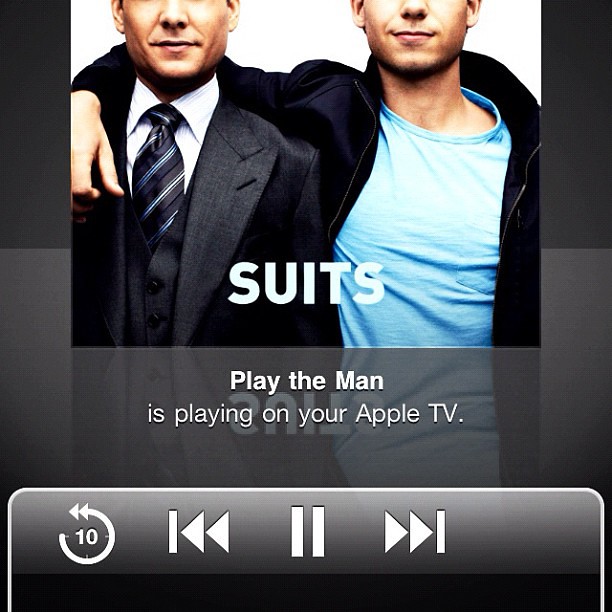The image appears to be a screenshot from an Apple TV interface, displaying a paused episode of the show "Suits" titled "Play the Man." The picture shows two Caucasian men from the nose down to the waist; the top part of their faces is cut off. The man on the left is dressed in a gray suit with a navy blue tie adorned with light blue diagonal stripes, paired with a white button-down shirt. The man on the right is wearing a black zip-up jacket over a blue t-shirt. Both men are partially cropped from the frame. Below the image, the interface includes playback controls, such as pause, fast-forward, rewind, and "skip back 10 seconds" options, indicating it is a streaming or multimedia control screen. The text on the screen reads, "Suits," and "Play the Man is playing on your Apple TV."